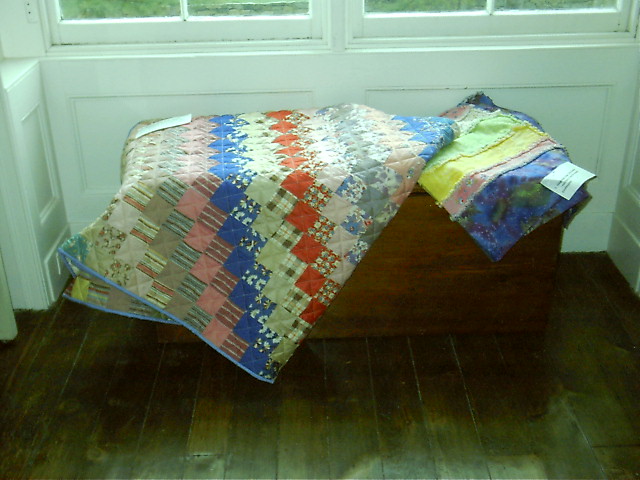In the image taken indoors, we see a room with white walls featuring two white-trimmed windows. The floor is composed of real wood, with dark and light boards mixed together. A medium brown cedar chest without feet sits directly on this wooden floor beneath the windows. Lying on top of the chest are two handmade textiles. The larger item on the left is a quilt with a blue border, adorned with various colored checkered designs including solid reds, blues, patterns with white flowers, stripes, and diamond shapes in blue, peach, coral, mint green, gray, brown, and beige. This substantial quilt, possibly king or queen size, is neatly folded. Next to it, on the right, is a smaller homemade textile, likely a pillowcase, characterized by layers of blue, yellow, pink, and green, with white frills. Both textiles have tags stitched onto them, hinting at their handcrafted origins.